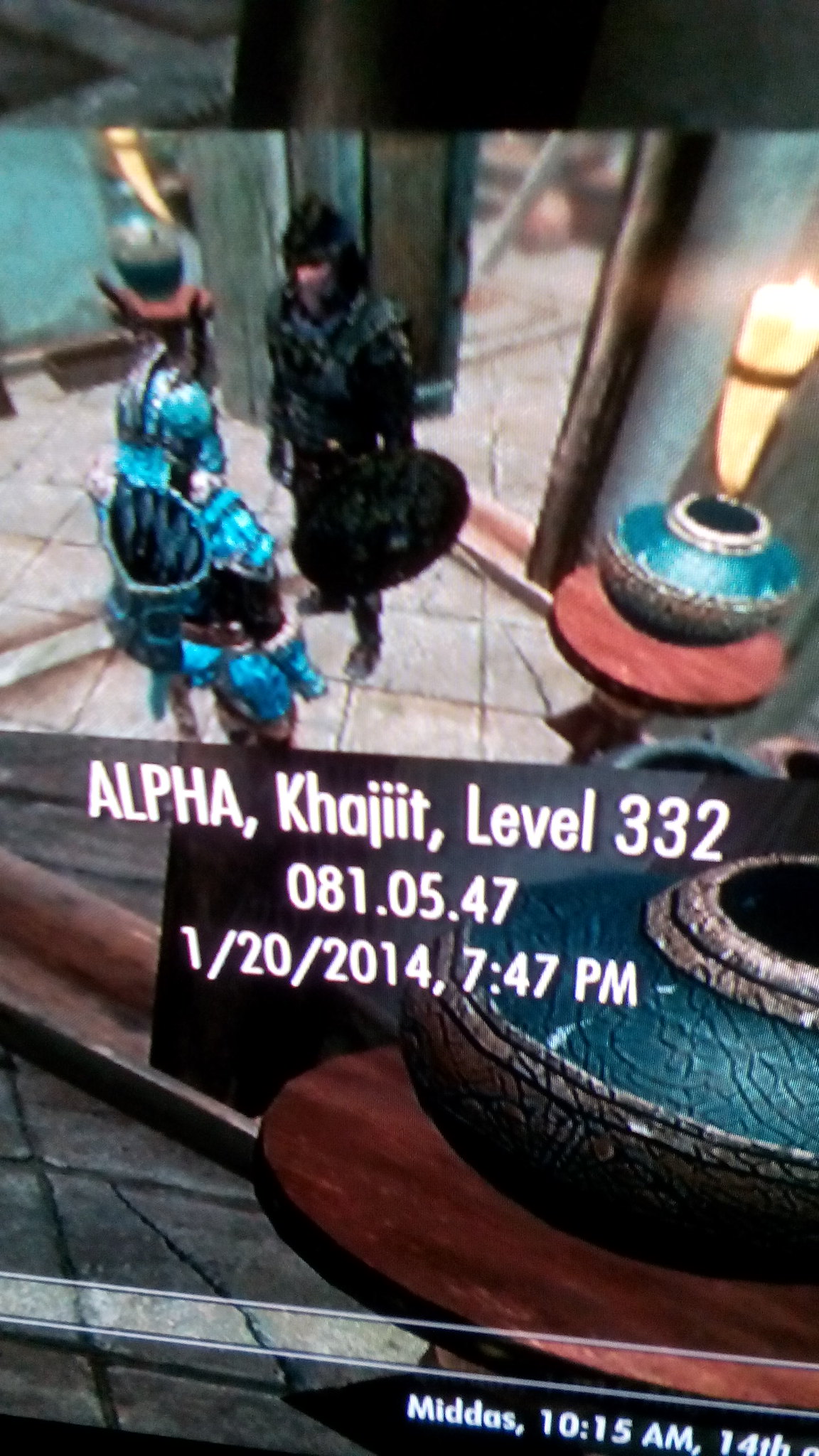The image is a detailed screenshot from the video game Skyrim, depicting a third-person perspective. At the top, it shows a small image with two armored characters standing face-to-face in a room with tile floors. The character on the left wears blue metallic armor and has a bow with a quiver on their back. On the right, another character dressed in black armor, is equipped with a round black shield and a helmet. Towards the bottom, there is displayed text including "Alpha Khajiit, Level 332, 081.05.47, 1-20-2014, 7:47 PM," likely indicating a saved game file. Additionally, a semi-transparent black overlay near the center reads "Alpha Khajiit, Level 332," confirming that this is during mid-game play. The scene also includes detail of the environment with a brown table and a blue vase positioned across from one another.